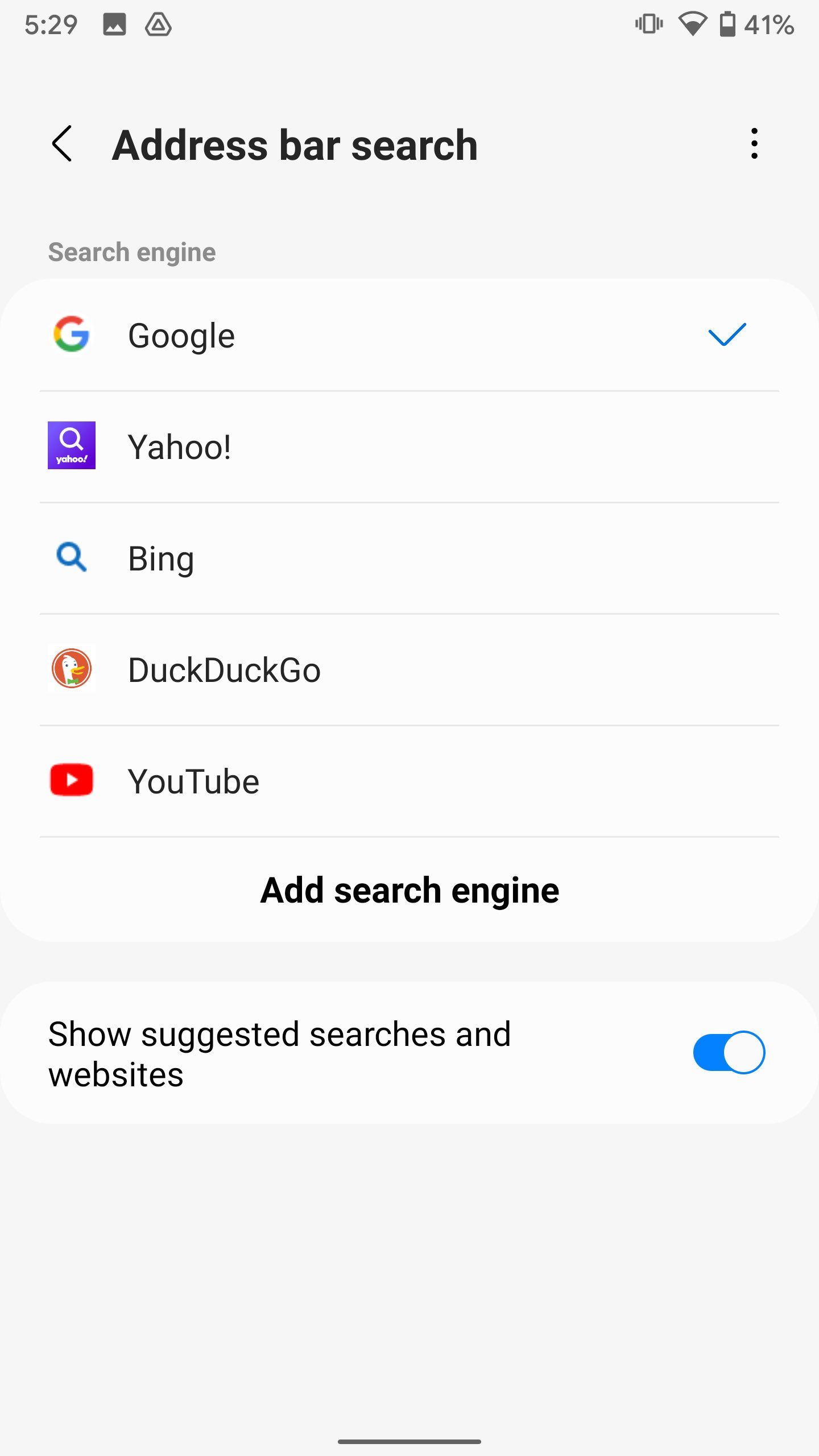A detailed screenshot displaying a smartphone screen at 5:29 PM with a battery life of 41%. The screen exhibits the interface of a browser or settings menu. At the top, a left-pointing arrow is situated next to a search bar reading "Address bar search." To the far right of this row, three vertically aligned dots symbolize additional options. Below, the browser settings indicate the preferred search engine: Google, marked by a blue checkmark. Alternative search engines listed include Yahoo, Bing, DuckDuckGo, and YouTube, followed by the option to add a search engine. An active toggle beside "Show suggested searches and websites" is apparent, highlighted in blue. The overall background sports a light gray hue, almost white, but discernibly gray in contrast with pure white. A subtle detail is visible at the bottom of the image: a short, one-inch long gray line centered at the bottom edge.